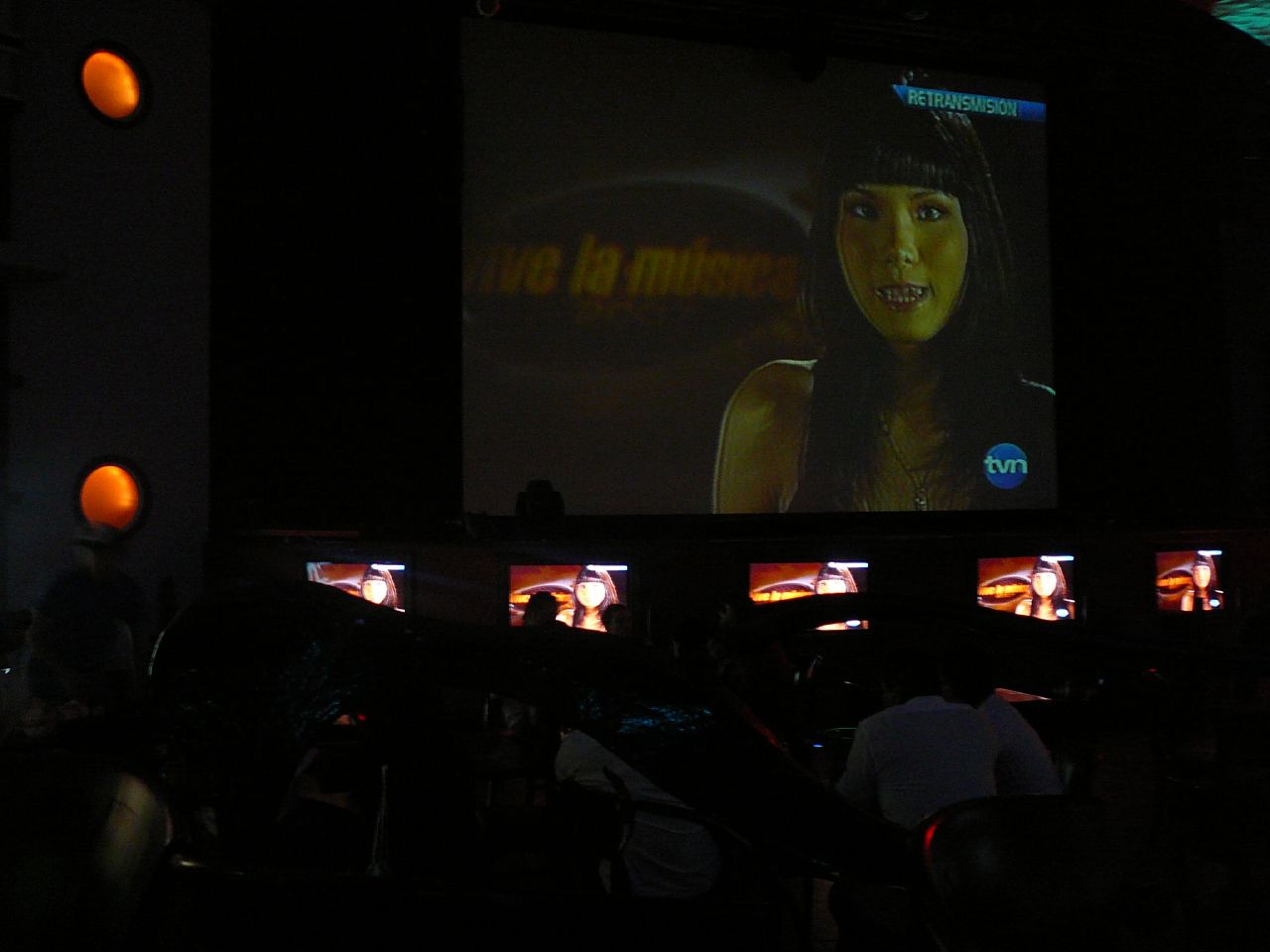The photograph depicts a dark room filled with about 15 to 20 people, many of whom are male and wearing white shirts, sitting and facing a series of monitors and a large screen at the front. The primary visual focus is a large screen displaying an image of a woman with her mouth open, smiling directly at the camera; she has long brown hair and a greenish skin tone, possibly due to the lighting or image quality. Surrounding the large screen are five smaller monitors that replicate the same image. The backdrop of the large screen features a logo in Spanish, "Viva La Musica," in an oval shape, and a "TVN" logo in the bottom right-hand corner. The room's darkness is punctuated by the light from the screens and a few circular lights on the wall, creating an environment that could be a bar, a nightclub, or a conference room. Despite the visual focal points, the purpose of the gathering remains unclear as most attendees are not actively watching the monitors.